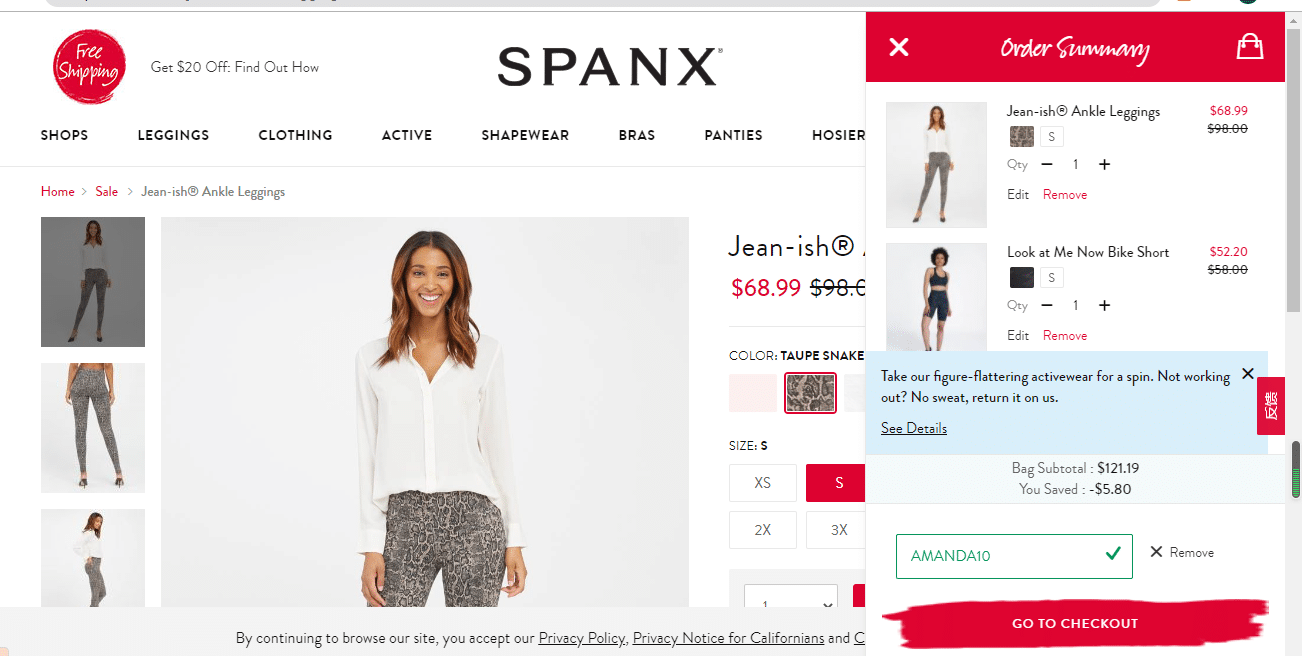This is a screenshot of a webpage from the online store Spanx. In the top-left corner, there is a red circle with white text that reads "Free Shipping." Next to it, there's a promotional note stating, "Get $20 off." 

The Spanx logo, displayed in bold text, is prominently featured above a navigation menu with the categories: Shops, Leggings, Clothes, Octaves, Shapewear, Bras, Panties, and Hosiery. Beneath this menu, a breadcrumb trail shows the user's navigation path: Home > Sale > Teenish Ankle Leggings.

On the left side, there are three smaller images displayed vertically. The top small image and the larger image to the right both feature the same woman modeling leopard print leggings paired with a white, long-sleeve shirt and a high-collared hairstyle. The second smaller image provides a close-up view of the leggings. The third smaller image shows the woman again in a side pose. 

To the right of the larger image, the product details are listed:
- Item: Teenish™ Ankle Leggings
- Price: $68.99 (reduced from $98)
- Color: Top Snake
- Size: Small

Alongside the product details, there's an expanded order summary section:
- Teenish™ Ankle Leggings: $68.99, Quantity: 1 (option to remove)
- Look At Me Now™ Bike Short: $52.20, Size: Small, Quantity: 1 (option to remove)

A promotional message below the order summary reads: "Take our figure-flattering activewear for a spin. Not working out? Not sweating it? Return it on us. See details."

The bag summary indicates a total of $121.19 with savings of $5.80. There is also a discount code "Amanda10" applied, with the option to remove it. A "Go to Checkout" button is displayed at the end.